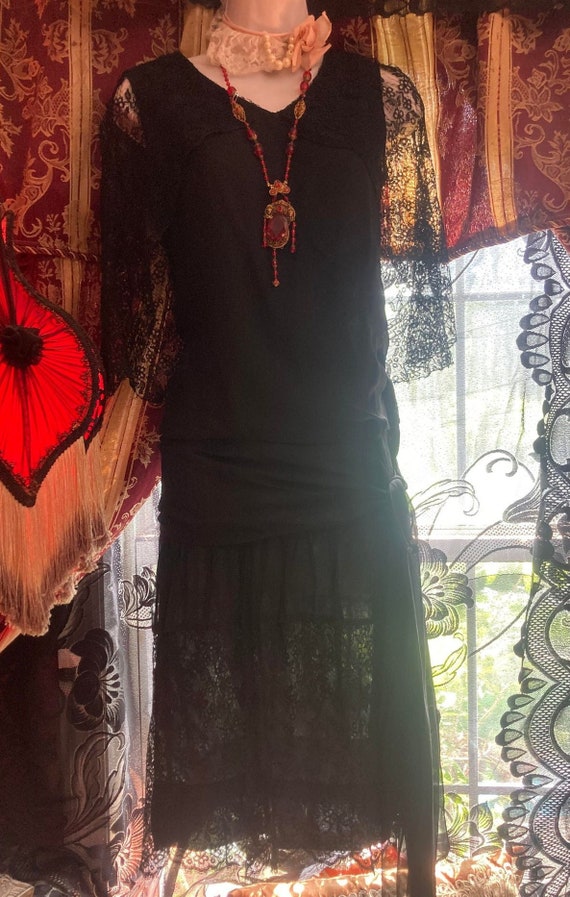The image captures a detailed view of a black dress displayed on a headless mannequin torso, situated in an indoor setting. The dress features delicate, laced sleeves and a skirt with a see-through pattern that starts midway down the legs, emphasizing its elegant filigree design. Draped around the mannequin's neck is an elaborate necklace adorned with red jewels or crystals, golden highlights, and numerous small beads. Additionally, a flowery neckband circles the mannequin's neck, adding to the ornate presentation.

The backdrop of the scene is a large window, partially covered by rich red material embellished with yellow floral designs at the top. The lower portion of the window is covered with black, see-through fabric, allowing a glimpse of the sunny outdoors and nearby greenery. To the left of the frame, a detailed red and black lampshade, decorated with golden tassels and shaped like flowers or leaves, adds a touch of handcrafted elegance to the room. The meticulous details of both the dress and the surrounding decor lend a sense of artisanal craftsmanship to the overall image.